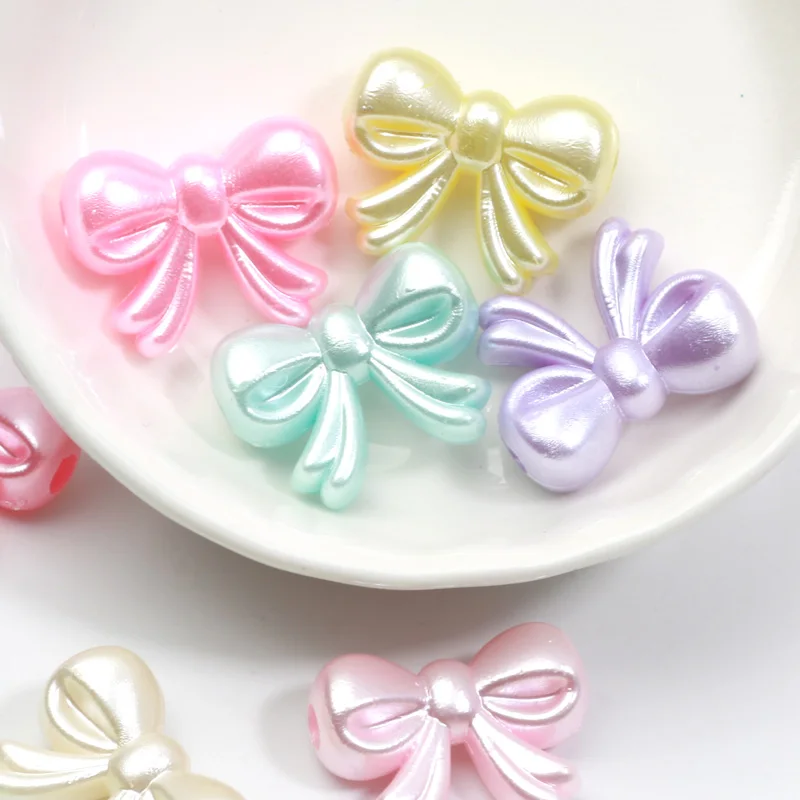The image features an assortment of small, vibrant bow ties, which appear to be decorative items made of plastic with a shiny, pearly finish. These bows come in a variety of pastel colors, including hot pink, light pink, purple, turquoise, Tiffany blue, gold, and a beautiful pearl color. While some bows are scattered on a white background, others are arranged inside a thin, pure white porcelain dish or ball that lies on a white surface. The bows, potentially for crafting or decoration, could be used to create children's jewelry or adorn other items with glue. The arrangement shows a pink bow at the top left, a yellow bow to its right, a light green bow below, and an upside-down purple bow beside them. Additional bows, including a light pink one, are positioned in front of and around the dish, contributing to the overall playful and colorful aesthetic of the scene.